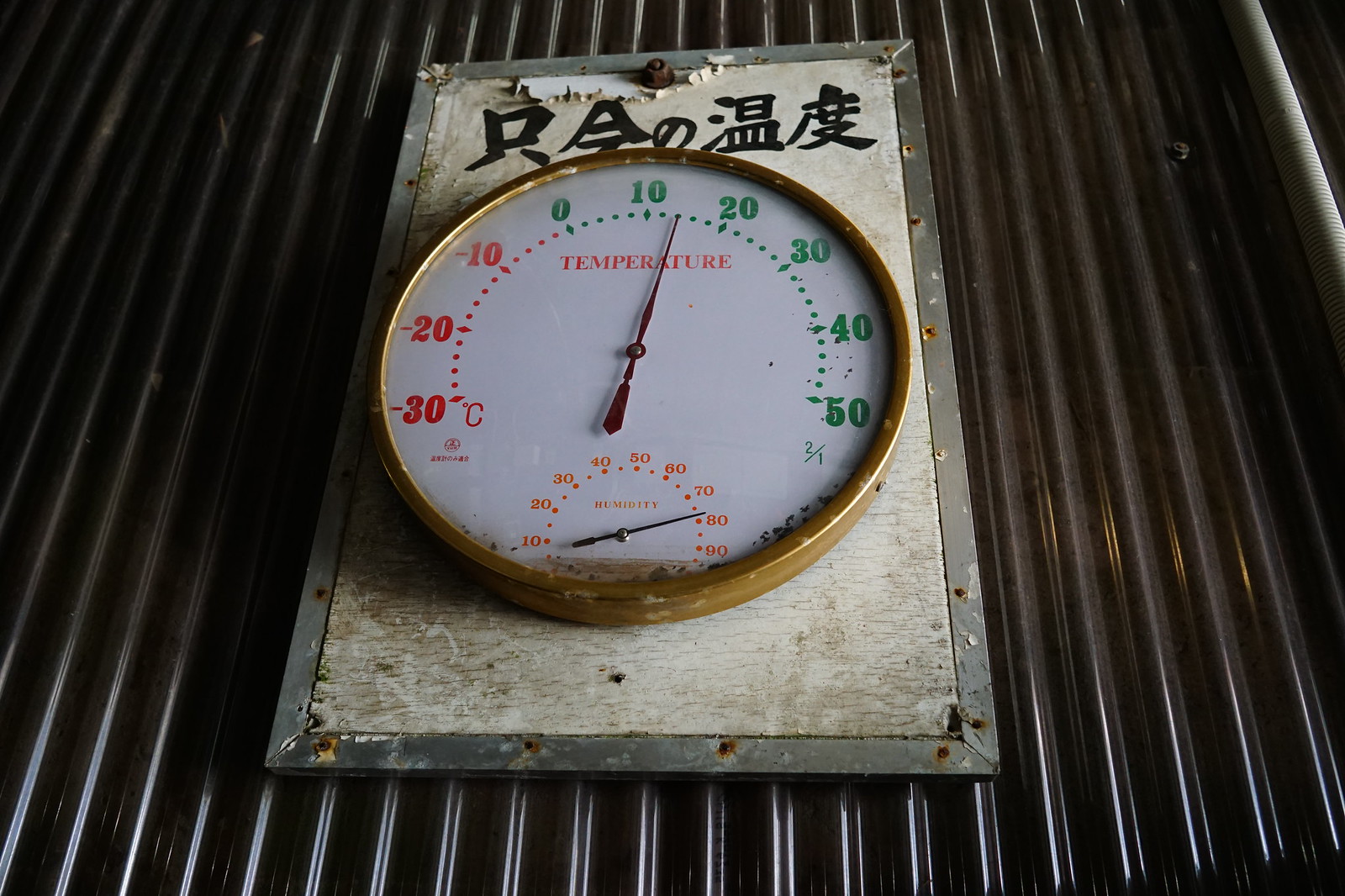A detailed image description:

This image features a temperature gauge prominently displayed on a white, oblong metal plate, which is surrounded by a metallic silver trim. The plate is mounted atop a black, ribbed tray made of a rubberized or plastic material. The tray is accented with silver-colored edges that frame the black ribs elegantly.

The temperature gauge itself is round and enclosed in a polished brass rim, adding a touch of vintage appeal. The gauge has a white face with large, clear numerals indicating temperatures ranging from -30 to +50 degrees Celsius. The boundaries of -10 through -30 degrees are marked in green, signifying extreme cold temperatures. The gauge needle currently points to approximately 13 degrees Celsius.

Positioned below the main temperature dial is a smaller subdial, which likely measures atmospheric pressure or humidity, though its specific function is not immediately clear. This subdial features numbers in a bright orange color and increments graduated in units of 10, with the indicator needle pointing just above the 75 mark.

At the top of the oblong metal plate, there are inscriptions in Chinese characters, suggesting either the origin of the device or its manufacturer. The overall scene is one of precision instrumentation, set against a contrasting background that highlights the functionality and aesthetic design of the temperature gauge.